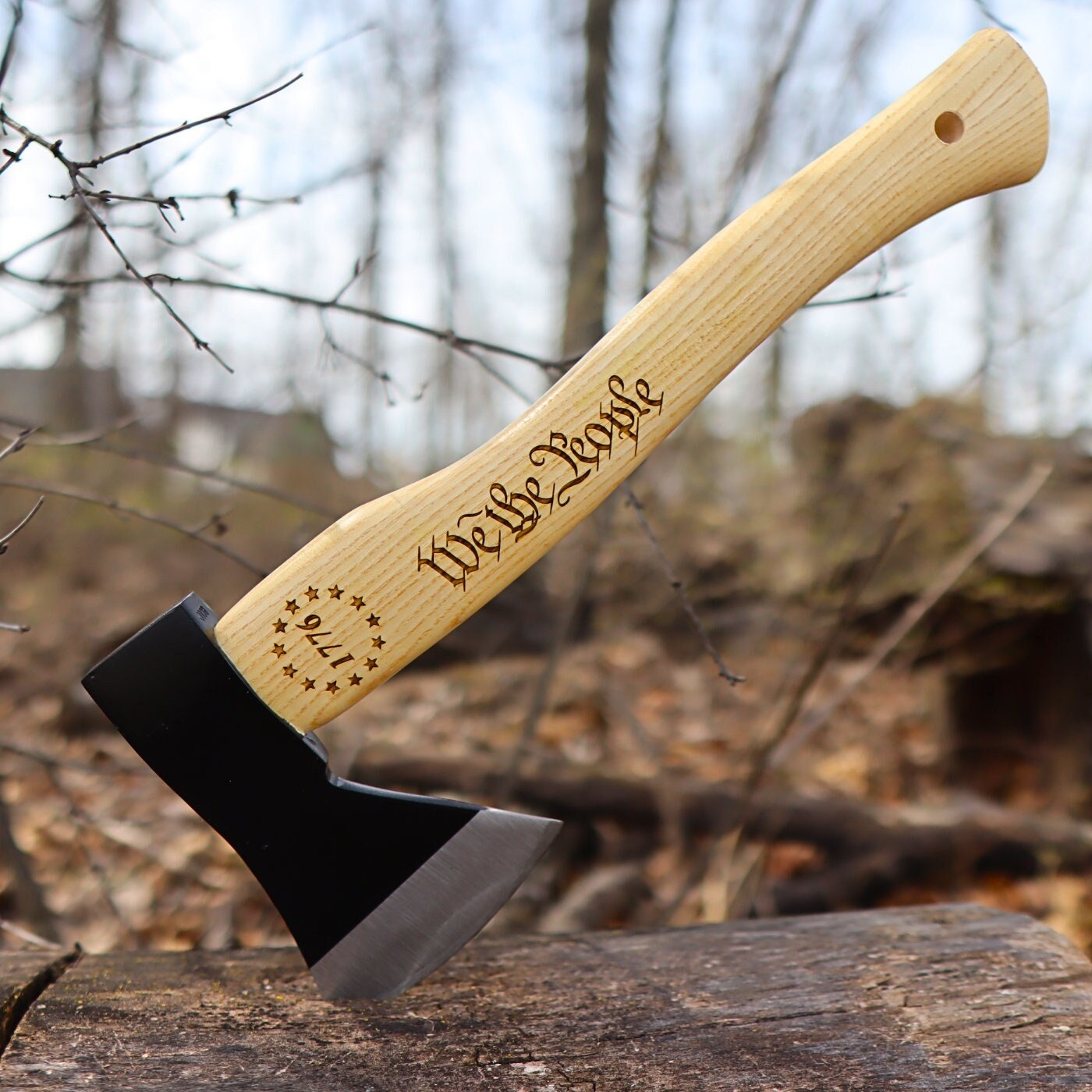The image captures a square photograph taken outdoors during the daytime, featuring a prominent axe embedded in a piece of wood. The handle of the axe, a light tan hardwood with horizontal stripes, stands upright with intricate details. At the top of the handle, "1776" is encircled by a ring of stars, etched into the wood, and mid-handle, the phrase "We The People" appears in script reminiscent of the U.S. Constitution. The axe head has a sleek black body and a sharpened silver blade edge, firmly lodged into the log. The background is a blurred forest scene filled with bare branches and fallen leaves, accentuating the axe's sharp focus. The wintry outdoor setting under a light grayish-blue sky suggests a serene yet solemn atmosphere.